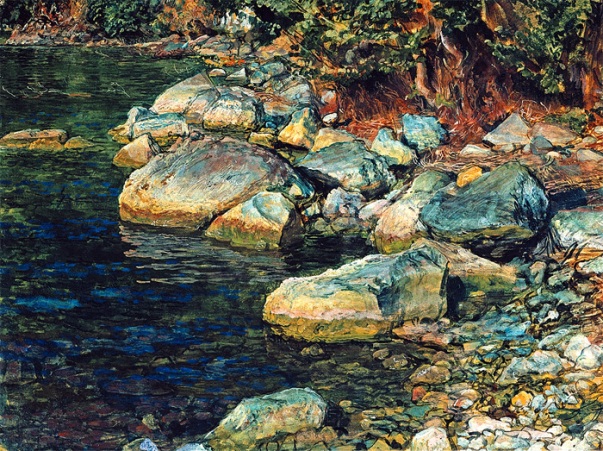The image, an intricate painting titled "Water and Stones" by Ivanov, depicts a serene shoreline of a pond with a harmonious interplay of rocks and water. On the right side of the painting, there is a collection of stones that start small and become progressively larger as they extend towards the center. These stones, predominantly white with patches of green moss, have subtle hues of blue and brown, creating a natural mosaic. The pond's water, located on the left side, is shallow enough to reveal the rocks at the bottom. Its surface, shimmering with shades of glossy blue and green, is gently rippled, reflecting the overhead rocks. In the upper right corner, tree roots and a rich red dirt base are evident, accompanied by green leaves that hang gracefully down from the tree, adding a touch of vibrant life to the composition.